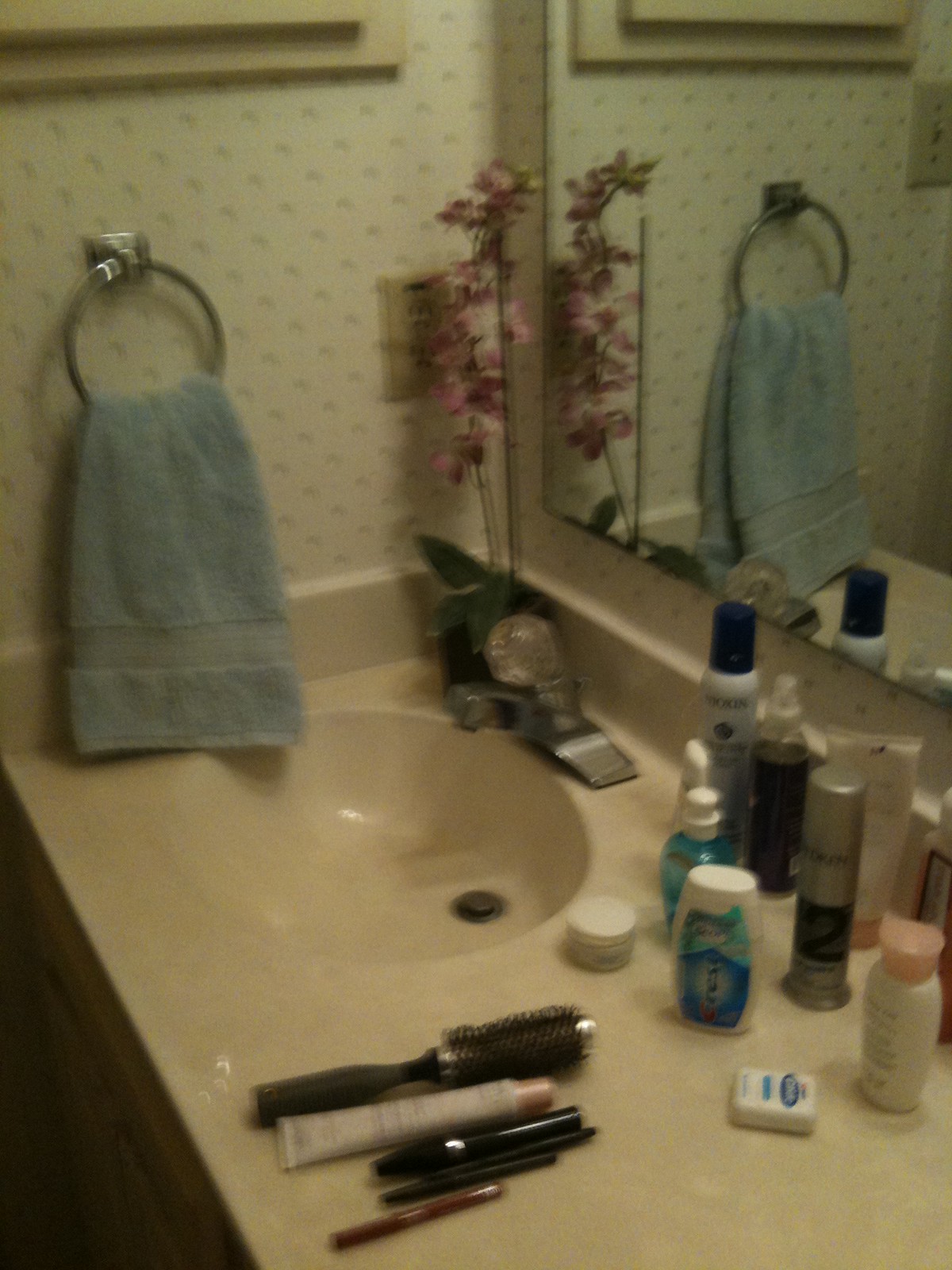This slightly blurry photograph showcases a bathroom countertop with a plethora of details. The wall in the background features a light polka dot or floral design, predominantly white. Just below hangs the lower part of a picture frame in a light wood or off-white color. Below this, a stainless steel ring towel holder supports a light blue hand towel. To the right of the towel holder, there's a tan outlet with two prongs.

Adjacent to the outlet, a cluster of pink orchids with long stems gracefully emerge from a dark green vase. The countertop itself, in off-white, hosts an array of personal care items including toothpaste, dental floss, shampoo, hairspray, a round brush, and makeup. A single-handle, steel-colored faucet with a plastic crystal knob for hot and cold water adorns the sink. The mirror above the sink reflects the arrangement of items, prominently featuring the flowers and the hand towel in its upper right section.